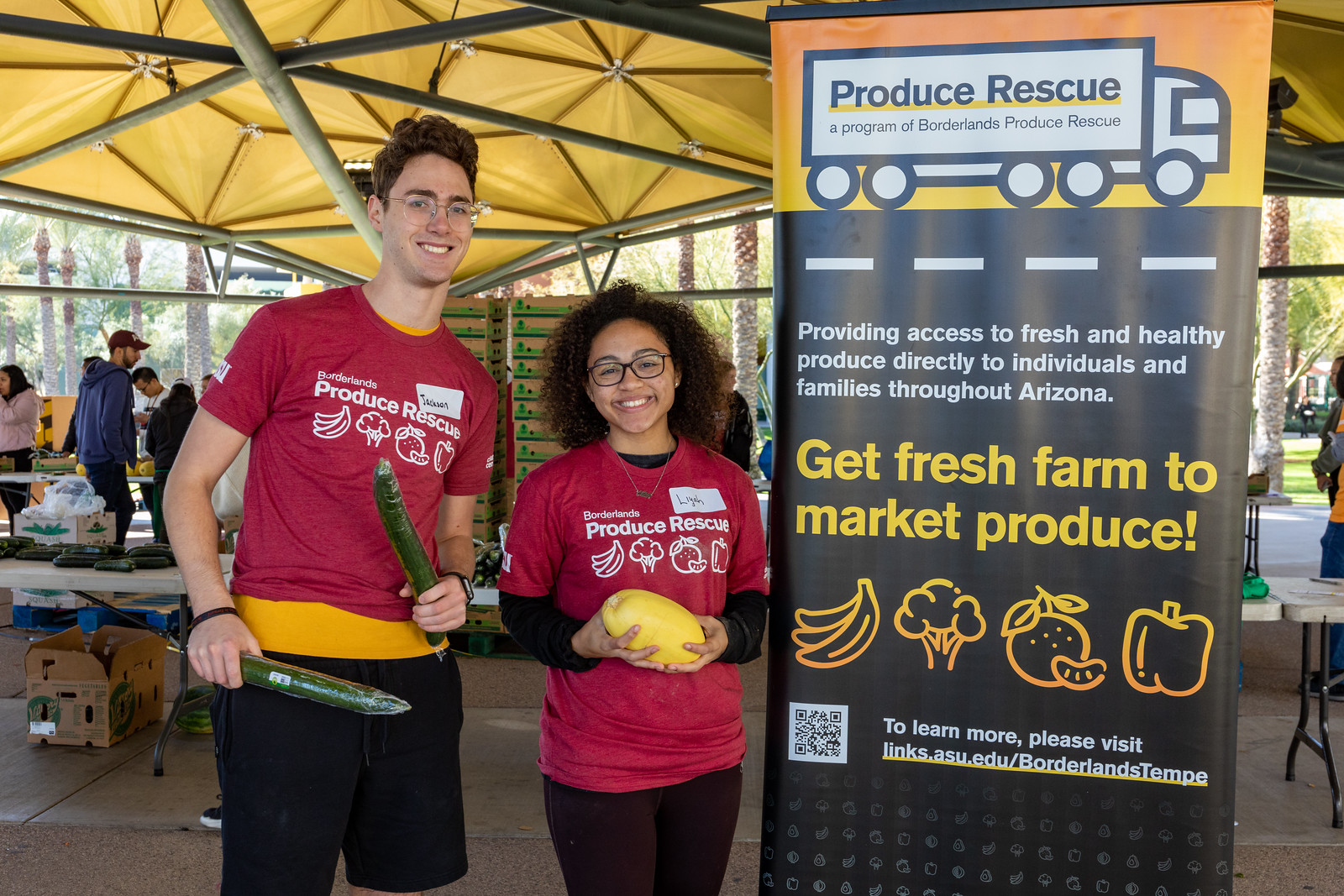In the image, we see an outdoor farmer's market set on a concrete ground surface, likely taken in the middle of the day. In the center of the image, there are two young individuals in their 20s, smiling and looking directly at the camera. Both are wearing red "Produce Rescue" shirts, with the young woman also donning black pants, curly hair, and glasses; she holds a yellow melon. The young man, wearing black shorts with a yellow band at the top, is playfully clinking two cucumbers together.

Behind them are tables displaying various vegetables, with people perusing the produce. On the left, there are more tables with cucumbers and a stack of boxes underneath. Above, a canopy tarp supported by poles provides shade.

To the right of the individuals is a sign that reads, "Produce Rescue, a program of Borderlands Produce Rescue, providing access to fresh and healthy produce directly to individuals and families throughout Arizona. Get Fresh Farm to Market Produce." The sign includes colorful illustrations of fruits and vegetables like bananas, cauliflower, apples, and peppers. In the background, we can also glimpse part of a hand-drawn truck on the sign, with further details and a website URL. The scene combines elements of community, healthy living, and access to fresh produce, framed by vibrant colors such as brown, black, yellow, red, gray, and green.